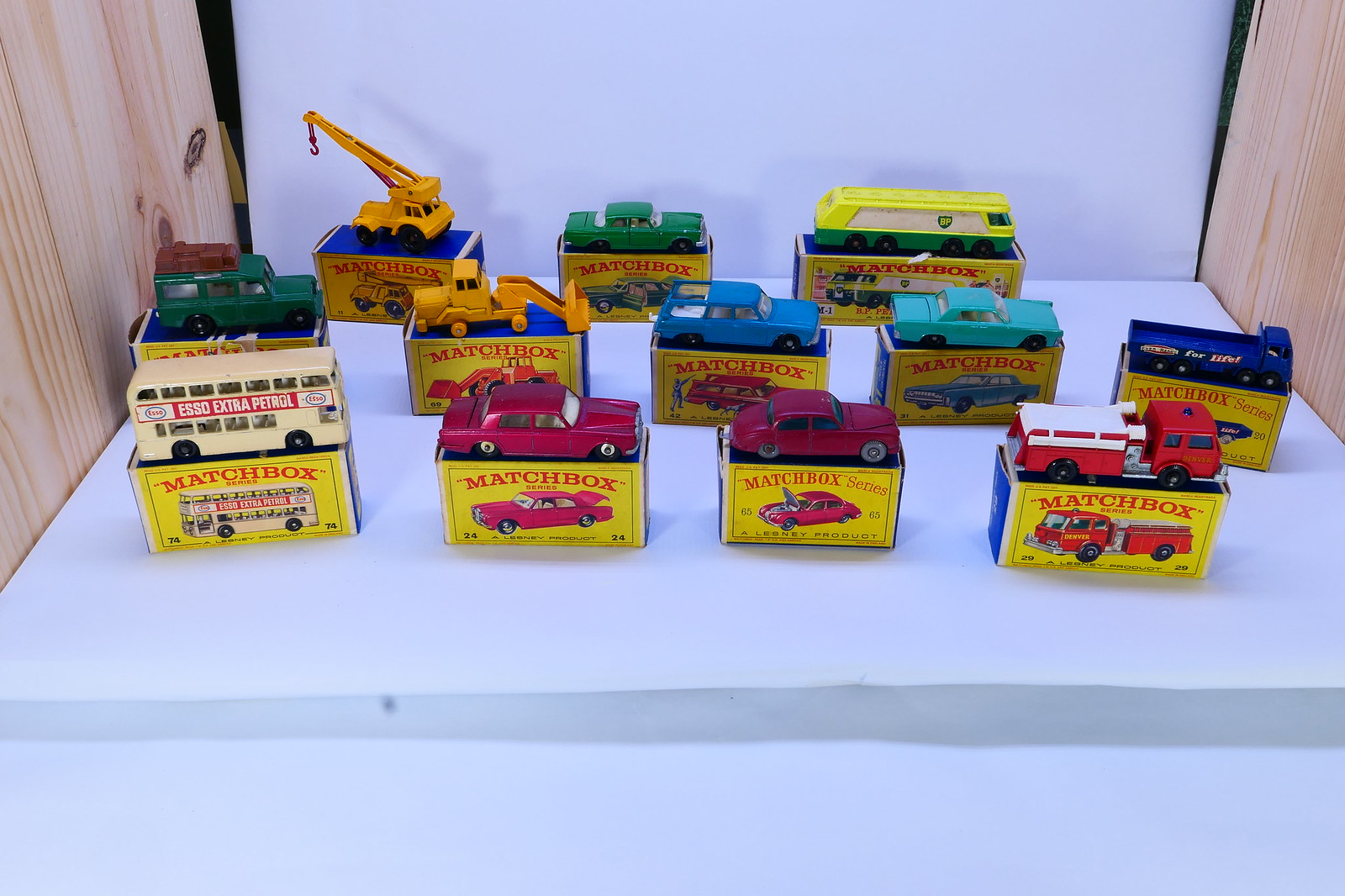This color photo showcases a detailed display of a vintage Matchbox car collection. Each vehicle, ranging from a fiery red firetruck and double-decker buses to various sedans and construction equipment, sits atop its original box. The boxes themselves feature a prominent yellow base with "Matchbox Series" written in red, complemented by a rich blue top adorned with specific numbers like 65, 24, and 69. Some vehicles, including a bus branded with "Esso Extra Petrol" and a couple of red sedans, remain notable. The background and ground of the display are stark white, possibly poster paper, accentuating the vibrant colors of the cars. Vertical wooden planks, likely unfinished pine, frame the sides of this thoughtful arrangement. The boxes include small text at the bottom that reads "a Lesney product," highlighting the authenticity and vintage appeal of the collection.